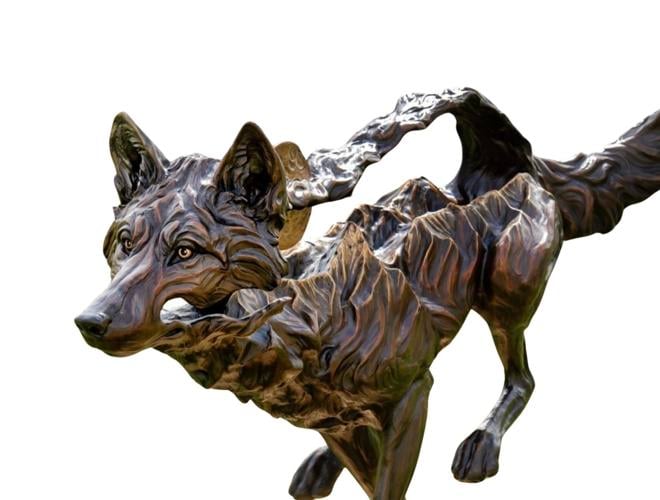The image depicts a meticulously detailed statue, possibly crafted from bronze or a type of dark and light mixed metal, featuring a wolf poised as if ready to leap. The sculpture showcases the wolf's realistic anatomical details, such as finely delineated ears, a forehead with expressive wrinkles, and pronounced legs and paws. The paws, intricately depicted, seem prepared to spring into action. The wolf’s body features ridges and a distinctive curvature stretching from the back of its head down to a slotted segment near its back leg, reminiscent of a coin's slot, rendered in a brass-like color. The wolf has haunting yellow eyes and a hollowed cheek, adding a spectral, ghostly quality to its visage. Along the wolf’s back is an artistic element that resembles a flowing stream or floating clouds, extending from the tail up behind the ears. A V-shaped support structure is visible under the front portion of the figure, contributing to the dynamic, almost ethereal presence of this striking sculpture.